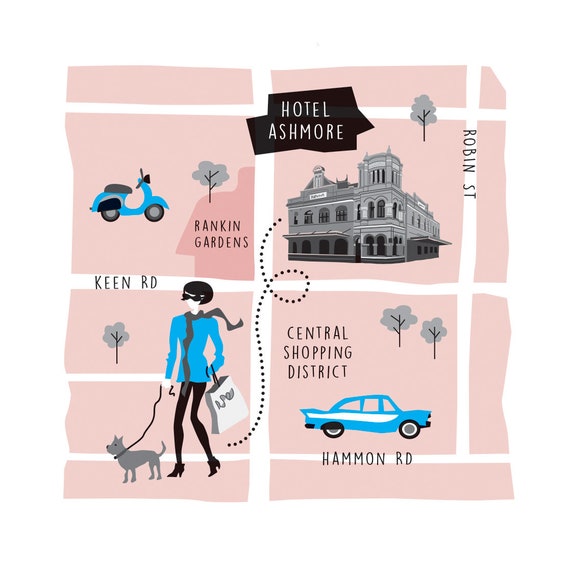This image is a stylized, cartoon-like city map predominantly in light pink with white roads depicted using negative space. The central feature, Hotel Ashmore, is located in the right-hand corner and is drawn in black and white. Surrounding the hotel, the map details several cross streets including Keene Road, Robbins Street, and Hammond Road. Scattered throughout are playful elements: a blue motorcycle near Rankin Gardens in the northwest, a distinctive blue car at the bottom, and the Central Shopping District with various dotted trees in the southeast.

Near the bottom, a detailed illustration shows a thin woman walking a dog on a leash, dressed in a blue jacket, black pants, black boots, and a gray scarf. She has short hair, black glasses, and is holding a bag. A dotted line swirls from her position up towards the hotel, indicating a path. The overall design is simplistic, likely intended for a brochure or city guide to provide engaging and easy-to-follow directions.